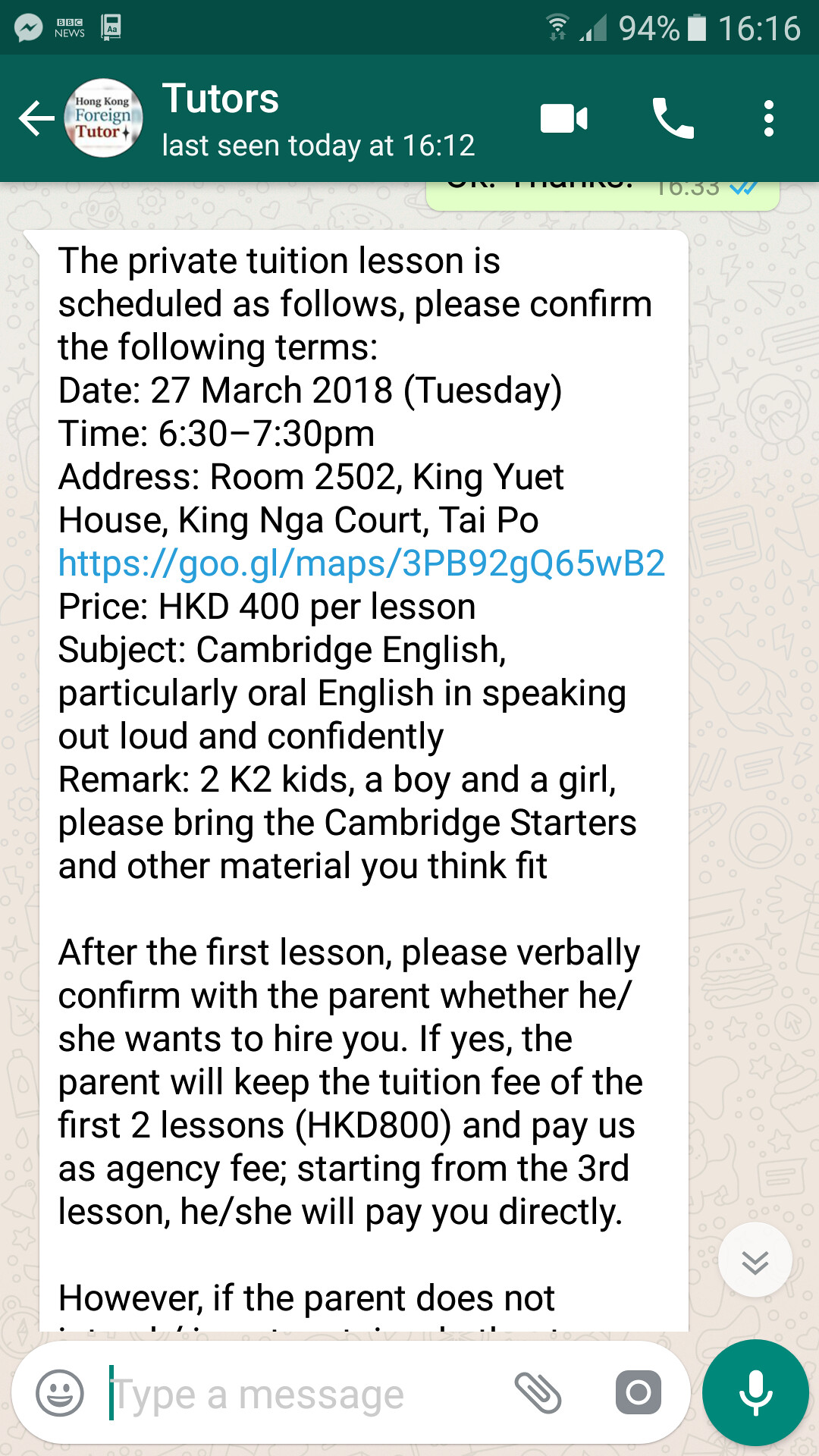This image is a detailed screenshot of a WhatsApp group chat on someone's phone. At the top of the screen, typical WhatsApp icons are visible on the left side, including the app's logo. On the right side, the device's information is shown, displaying a signal strength icon, a battery percentage at 94%, and the current time of 16:16, all in white font against a deep forest green background.

Below this, information about the group chat named "Tutors" is displayed on a slightly lighter green background. To the left, there's a back arrow icon, followed by a circular profile picture labeled "Hong Kong Foreign Tutor," although only partially visible. To the right of the profile picture, the group name "Tutors" is clearly written with a status below indicating "last seen today at 16:12." Adjacent to this, there are icons for video chat, a phone call, and three vertically aligned dots indicating more options.

The main content of the screenshot shows a message in a white background with predominantly black text. The message details are as follows: The private tuition lesson is scheduled with terms including the date, 27 March 2018 (Tuesday), and the time, 6:30 to 7:30 PM. The lesson's address is Room 2502, King Yuet House, King Nga Court, Tai Po. A Google Maps link is also included, highlighted in blue. The tuition cost is HKD 400 per lesson. The subject is Cambridge English, focusing particularly on oral English and speaking confidently. The lesson involves teaching two kids, a boy, and a girl, who are expected to bring Cambridge Starters and other relevant materials. Post the first lesson, the tutor is to verbally confirm with the parent if they wish to continue the tuition, after which the parent will retain the tuition fee for the first two lessons (HKD 800) as an agency fee. From the third lesson onward, payments will be made directly to the tutor. The message is partially cut off, ending with the line, "However, if the parent does not..."

Overall, the image gives comprehensive details about a scheduled private tuition session in a WhatsApp group chat format.